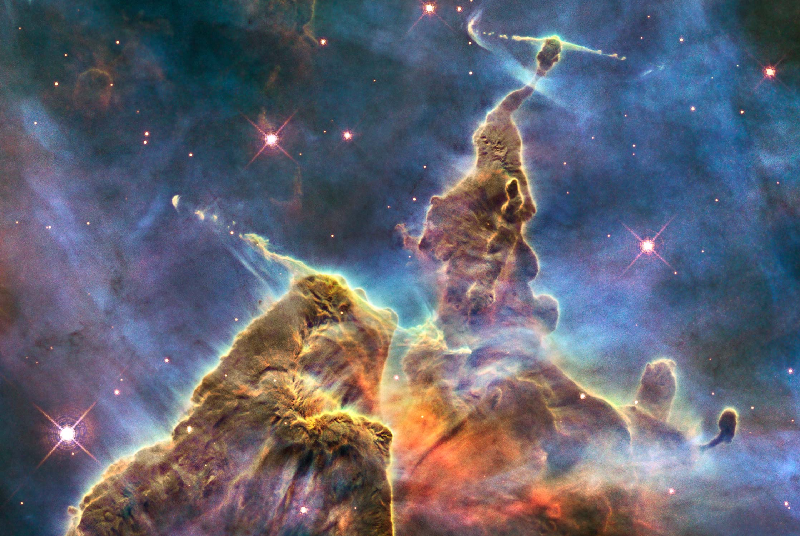The photograph is a richly detailed deep space scene, likely captured by the Hubble telescope or a similar device, featuring vibrant and cloudy nebulas in shades of bright golden, yellow, and orange, intermixed with greenish and blue hues, and dotted with purple clouds. Bright, gleaming stars of varying sizes pepper the image, accompanied by numerous smaller star dots. Central to the scene is a striking, otherworldly formation resembling a mountain or large boulders, with an orange light radiating from its core. Topping this structure is an intriguing oval-shaped object emitting light in a horn-like pattern, contributing to the intergalactic ambiance of the image. Despite the surreal and fantastical elements, such as the interstellar formations and computer-generated feel, the photograph encapsulates a breathtaking and seemingly fictional solar system setting, complete with a dark, star-studded sky and white wispy clouds.